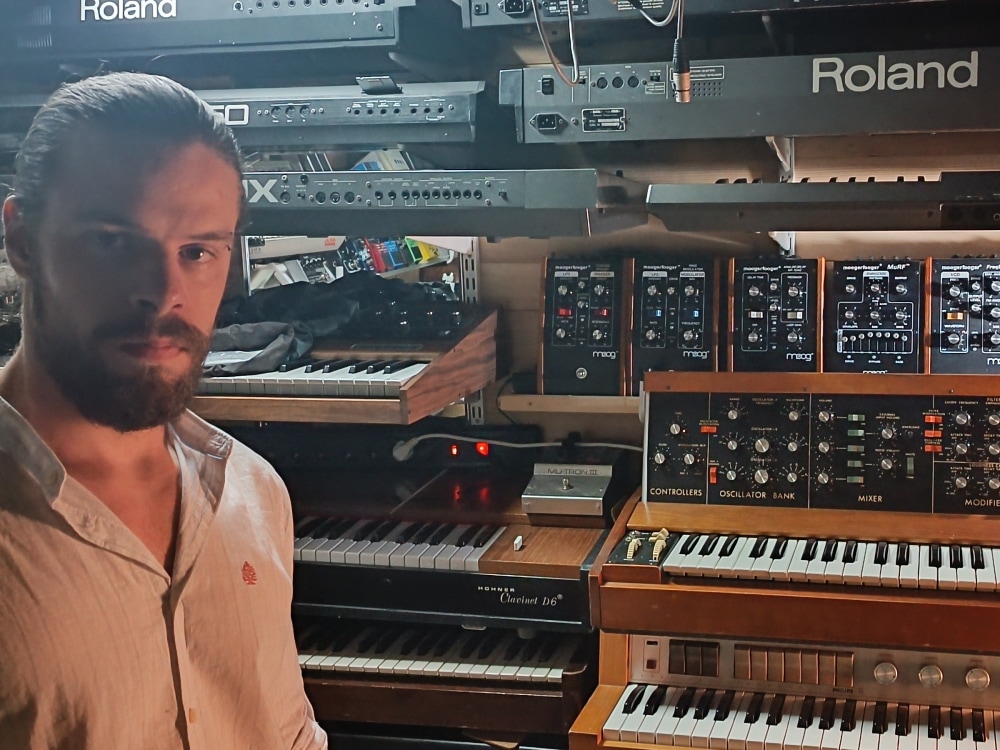The photograph features a white male, likely in his thirties, who appears to be a sound engineer or musician. He is positioned near the top-left corner of the image, wearing a white collared shirt with a red label on the left breast area. His shirt is unbuttoned at the top, revealing a casual look. He has brown hair that is slicked back, possibly into a ponytail, along with a full, neatly trimmed beard and mustache. He is staring intently into the camera.

The rest of the image is dominated by a variety of musical equipment, primarily keyboards and sound engineering devices. To the right of the man, there are five keyboards, with two on the right being made of wood. The top wooden keyboard has a brown wood finish and is marked with labels like "Controller," "Oscillator Bank," "Mixer," and "Modifier" in gold text. It prominently features the brand name "Moog," known for high-quality synthesizers, and is covered in silver knobs and red buttons.

On the left side of the image, there are three additional keyboards. One has a lighter brown wood finish with a silver box on it, while another, right below it, has a darker brown wood finish. There's also a black metal keyboard labeled "Clavinet D6," which features the words "Hohner" and "High" in white text.

Scattered across the background, various pieces of sound and musical equipment are visible, with several panels filled with knobs and buttons designed for audio manipulation. The brand "Roland" is noticeable on several devices, identified by the distinctive white lettering. Additionally, there are numerous cables and plugs, some of which are connected to the equipment, contributing to the complex and technical ambiance of a professional music studio.